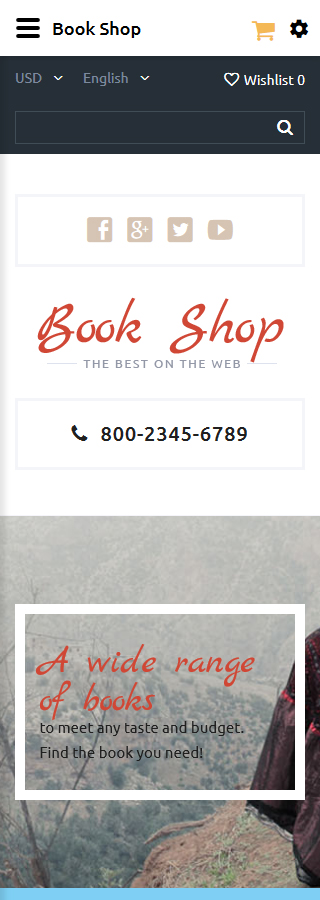This is a vertically oriented image taken from a smartphone, likely showing a screenshot of a website. 

The image features a white background, possibly illuminated by a computer screen. In the top-left corner, there are three thick horizontal black lines, which suggest a clickable menu for additional options. Adjacent to this, in bold black text, the words "Book Shop" are prominently displayed. On the top-right corner, a yellow shopping cart icon is visible, followed by what appears to be an account or settings icon.

Below this section, on the left, a black or gray rectangular box displays selectable options in white text: "USD" with a downward arrow, "English" with a downward arrow, and a heart icon. On the corresponding right side, the text "Wish List: 0" is shown. Centrally located beneath this, there is a small rectangular search bar with a white magnifying glass icon.

Further down, the background remains predominantly white, featuring a gray rectangular box housing social media icons for Facebook, Google Plus, Twitter, and YouTube. Directly beneath these icons, in red text, is "Book Shop," followed by the tagline "The Best on the Web." 

Below this section, another box provides a phone number, offering contact details. Descending further, there is an image depicting an outdoor scene with mountains and trees, stated within a wide white border. The text within this box reads: "A wide range of books to meet any taste and budget. Find the book you'll need."

At the very bottom of the image, a thin blue line completes the screenshot, visually separating the various sections.